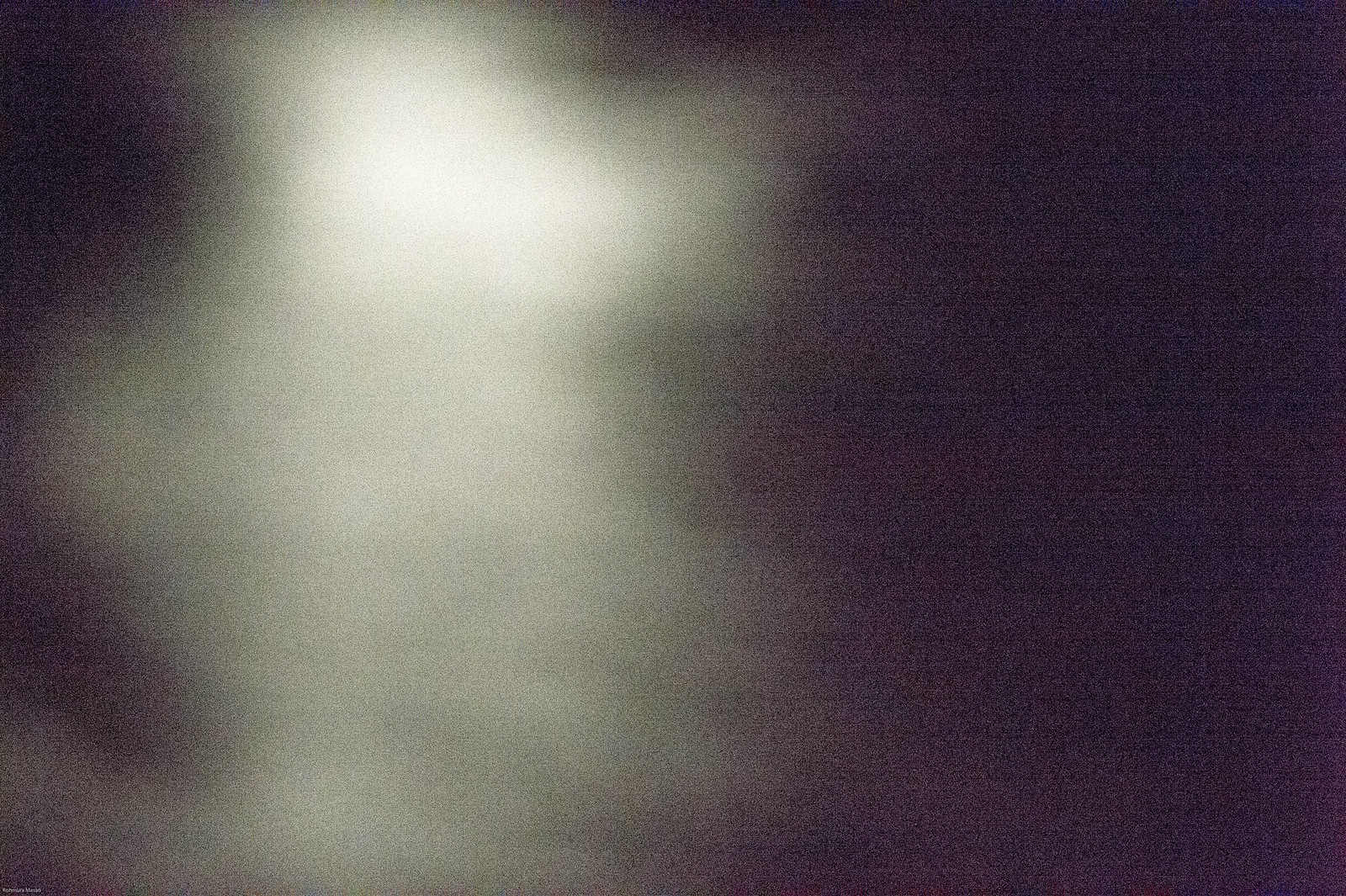The image is a highly blurry and grainy photograph in landscape orientation. Dominating the right side of the image is a very dark, brownish-black area that extends unevenly towards the left. This darker region transitions into a lighter area, characterized by a large, diffuse light spot that spans from the bottom to the top of the image. The light spot appears somewhat swirly and is most pronounced on the left side, giving the impression of irregular shapes; some might describe these shapes as vaguely resembling an arm or even a blurred white skull. To the far left, particularly at the top and bottom corners, the image fades back into darkness, reinforced by black areas that hint at an artificial light source, possibly emanating from a lamplight or similar. The overall graininess and indistinguishability of objects suggest it might be an unsuccessfully developed Polaroid or a photo taken at night, with reflective and wispy elements giving a smoky, shadowy appearance that ultimately merges into the pitch-black right side of the image.